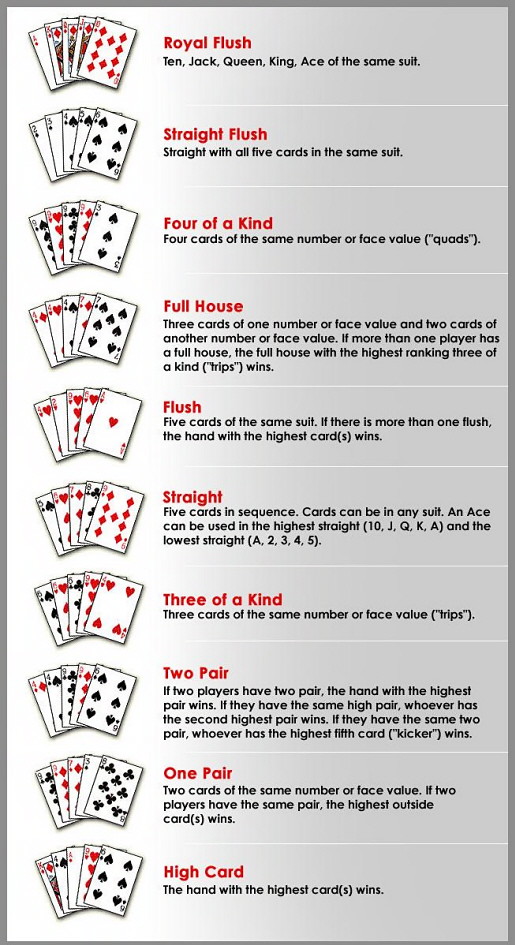This image provides a detailed explanation of poker hands and their rankings. It is illustrated with the following poker hands:

1. **Royal Flush**: A hand containing the 10, Jack, Queen, King, and Ace of the same suit. This is the highest possible hand in poker.
   
2. **Straight Flush**: Five consecutive cards of the same suit. For example, 5-6-7-8-9 of hearts.

3. **Four of a Kind (Quads)**: Four cards of the same rank. For instance, four Queens or four 7s.

4. **Full House**: Three cards of one rank and two cards of another rank. For example, three Kings and two 5s. If multiple players have a full house, the one with the highest ranking three of a kind wins.

5. **Flush**: Any five cards of the same suit, not in sequence. If there's more than one flush, the higher card wins. For instance, A-10-8-6-3 of diamonds.

6. **Straight**: Five consecutive cards in any suit. The Ace can be high (10, Jack, Queen, King, Ace) or low (Ace, 2, 3, 4, 5).

7. **Three of a Kind**: Three cards of the same rank. For example, three Jacks.

8. **Two Pairs**: Two sets of pairs. If two players have the same high pair, the one with the highest second pair wins. If the second pairs are also the same, the highest fifth card (kicker) decides the winner.

9. **One Pair**: Two cards of the same rank. If two players have the same pair, the highest outside card wins.

10. **High Card**: When no other hand is made, the hand with the highest card wins. For example, Ace-high.

The image serves as a comprehensive guide to understanding poker hand rankings and how to determine the winning hand based on different scenarios.